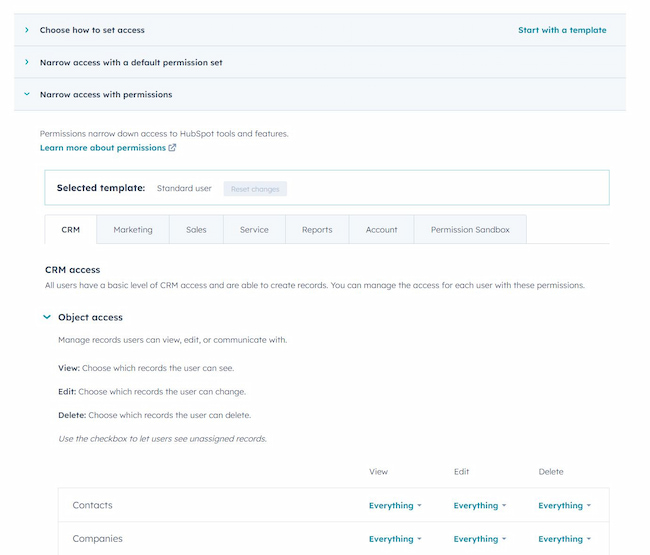**Caption:**

The image displays a detailed section of a website dedicated to setting user permissions. At the very top left, there is a rectangular box featuring a right-pointing arrow accompanied by the text "Choose how to set access." On the top right, there is an option highlighted in blue that reads "Start with a template." 

Below this, another right-pointing arrow guides users with the instruction, "Narrow access with a default permission set." Further down, a downward-pointing arrow offers the option "Narrow access with permission."

Next, there is a segment describing permissions: "Narrow down access to HubSpot tools and features." This portion also includes a green-highlighted link encouraging users to "Learn more about permissions."

The middle section, titled "Selected Template," displays the term "Standard User" in a light font, adjacent to a gray box labeled "Reset Changes."

Beneath, a series of menu tabs are visible, each tagged with specific sections: CRM, Marketing, Sales, Service, Reports, Account, Permission, Sandbox, with the CRM tab highlighted. The "CRM Access" section includes a comprehensive sentence explaining access details. The "Object Access" subsection follows, comprising five lines of information. 

A table with three columns and two rows is shown, where the rows are titled "Contacts" and "Companies," and the columns are labeled "View," "Edit," and "Delete." Each cell in the table features a drop-down arrow for further selection adjustments.